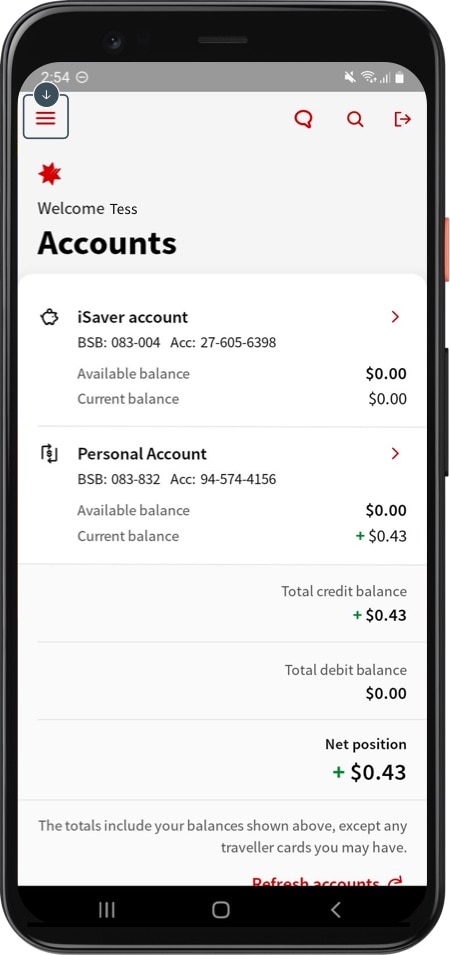In the image, we see a black mobile phone with rounded edges. The device features two buttons on its side: an orange button situated closer to the top and a longer black button below it. At the top of the phone, slightly left of center, is a small camera, alongside a rectangular speaker located in the center of the upper edge.

The phone’s screen displays an open banking app. The interface shows a red 'burger' menu icon at the top left, followed by a chat bubble icon, a magnifying glass icon, and a proceed or enter icon. Below these, the screen reads, "Welcome, Test Account."

The app lists two accounts:
1. **iSaver Account**
   - Available balance: $0.00 
   - Current balance: $0.00

2. **Personal Account**
   - Available balance: $0.00 
   - Current balance: +$0.43 (43 cents)

At the bottom, the app summarizes the financial status:
- **Total Credit Balance:** $0.43 (43 cents)
- **Total Debit Balance:** $0.00
- **Net Position:** +$0.43 (43 cents)

The detailed display on the mobile phone captures the intricacies of the user’s banking app interface, summarizing the account balances and overall financial position efficiently.